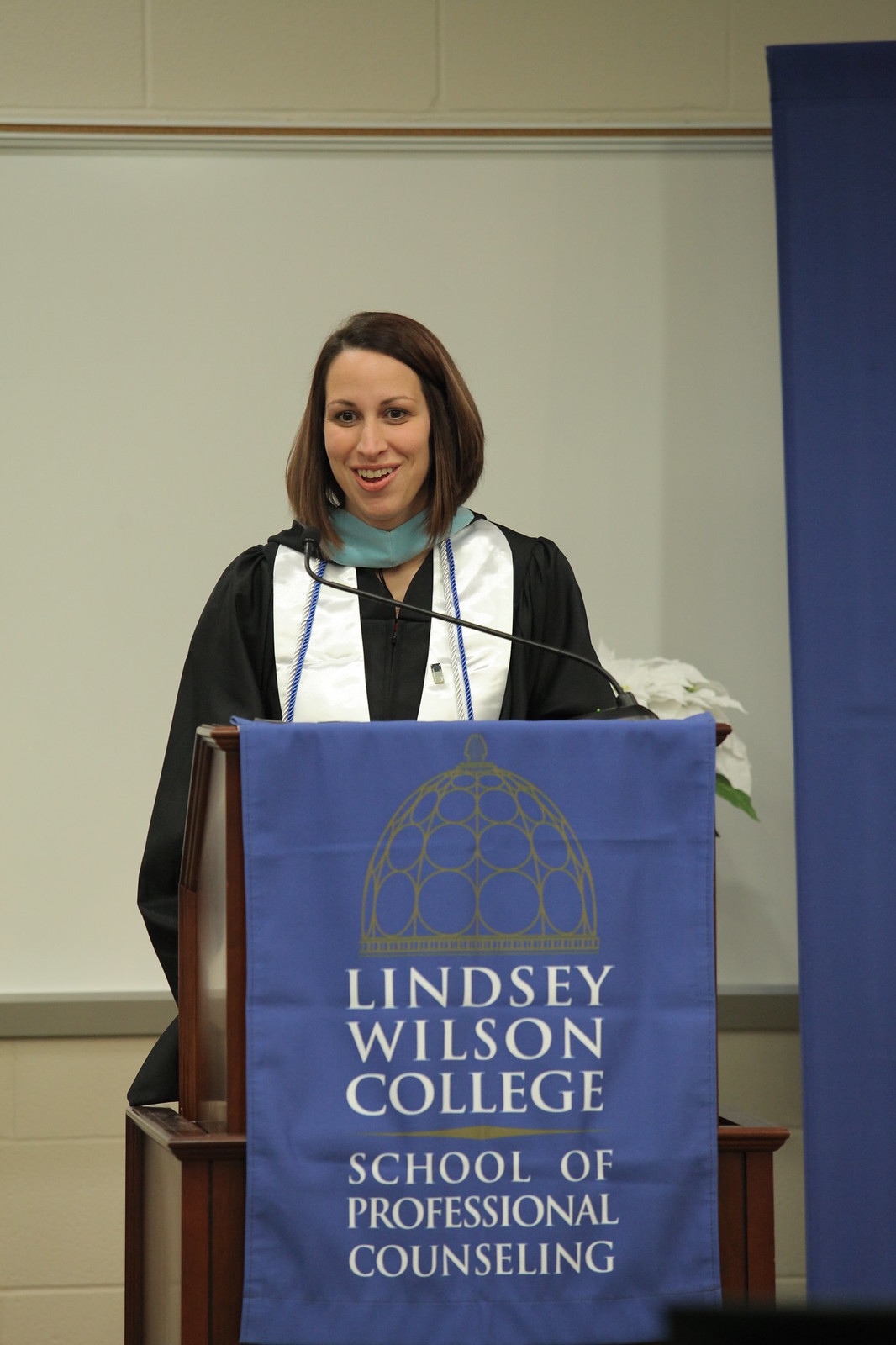The image depicts a woman, likely a Caucasian female with short brown hair styled in a bob, standing at a wooden podium adorned with a blue banner that reads "Lindsay Wilson College School of Professional Counseling" accompanied by a stylized drawing of a dome. The woman is dressed in a black graduation robe with white lapels, complemented by a teal-colored scarf or regalia and a long blue cord around her neck. She stands in front of a large white board, possibly within an auditorium or theater, addressing an audience, evidenced by her smile and the microphone positioned close to her mouth. Behind her, a partial view of a flower arrangement adds to the ceremonial atmosphere, suggesting that she is likely delivering a significant speech, such as a graduation address or a guest lecture.